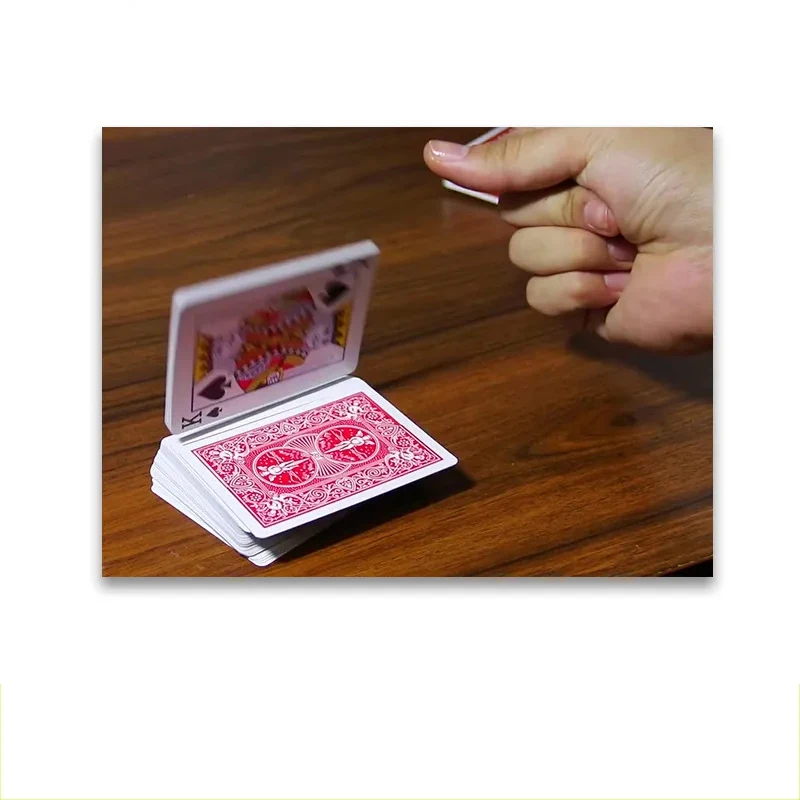The image showcases a person's right hand positioned in the upper right-hand corner, holding a small metal object with fingers partially curled. The hand is just visible and is cut off at the palm. Below, a dark brown, shiny table serves as the backdrop. To the left, a red-backed Bicycle brand deck of cards is featured, appearing to be in mid-shuffle. Approximately the top 10-20 cards have been flicked upwards at a 90-degree angle, and the king of spades is prominently displayed facing the camera. The capture suggests movement, as if the cards were just lifted or dropped, caught in action to create a magical, floating effect.